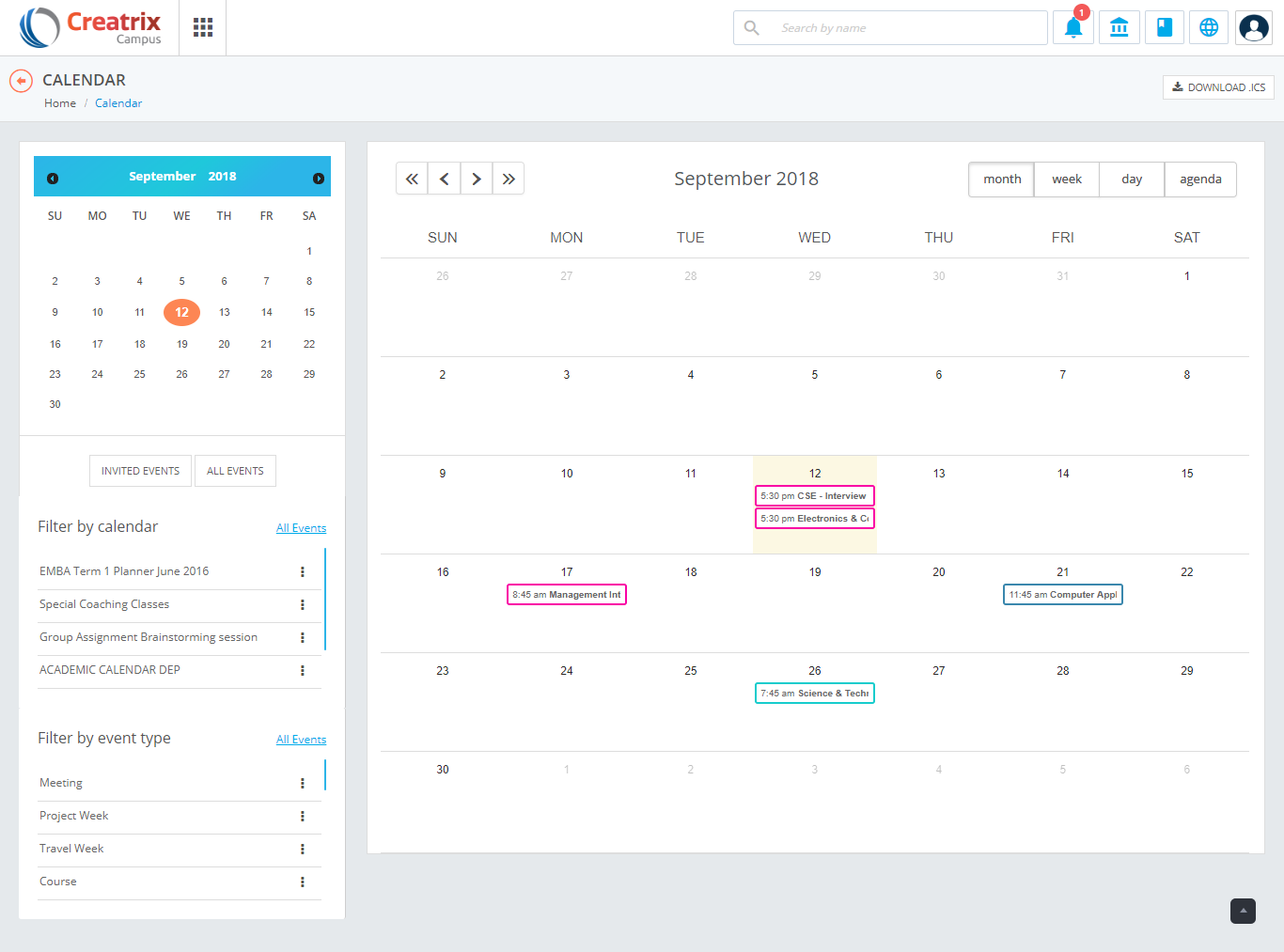In the upper left corner of the image, there is a partially filled circle. Inside the circle, the word "Creatrix" is displayed in bold orange text, spelled out as C-R-E-A-T-R-I-X. Directly below this, the word "Campus" appears in a similar orange font. Beneath these words is a search bar.

To the right of the search bar, there is a blue bell icon with a small red circle on its top-right corner containing the number "1". Adjacent to this, there is an image of a blue building. Next to the building, there is an icon that looks like a blue piece of paper or disc. Following this icon is a silhouette of a person enclosed in a square frame.

Towards the left side of the image, there is a calendar displaying "September 2018". An orange circle highlights the date "Wednesday, the 12th". The following messages on the calendar are outlined in a rectangle: Wednesday, the 12th; Monday, the 17th; and Wednesday, the 26th. 

Furthermore, to the left, the calendar shows options to "Filter by calendar" and "Filter by event type." This section allows users to customize their calendar view.